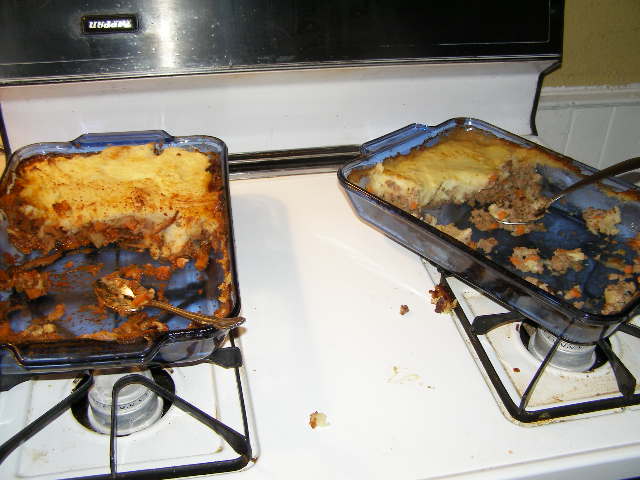This is a photograph of a vintage 1970s white gas stove with black grates, located inside a kitchen. The stove features four burners, evenly spaced in two rows. The backsplash is divided into two sections, with the top part being black and adorned with some indistinct white text, and the bottom part consisting of white vertical wooden paneling underneath a mustard yellow painted wall.

On top of the stove are two Pyrex glass casserole dishes, each placed on a separate row of burners. Both dishes are similar in size, approximately 9x11 inches, and each contains a large stainless steel spoon. The casseroles appear to be dinner dishes, one possibly resembling lasagna with a yellow melted cheesy top, and the other potentially a meat-based dish with a creamy white topping that could be either custard or mashed potatoes. The contents of both dishes have been significantly consumed; the dish on the left has half of its contents remaining, while the one on the right has only about a quarter left.

The overall setting suggests a cozy, somewhat dated kitchen scene, with the casseroles likely being shepherd's pie or moussaka, hinting at a hearty, communal meal that has been enjoyed.